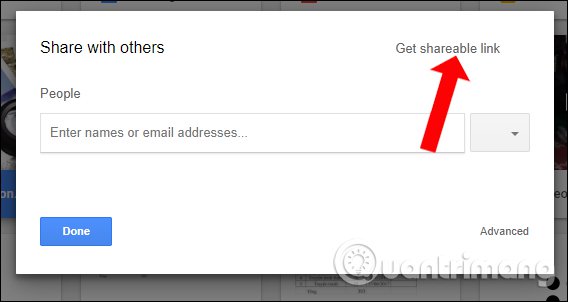The image is a screenshot of a Google sharing interface pop-up. The pop-up allows users to share content, visible in the background, which appears to be a webpage with photos. Prominently, a red arrow points to a button labeled "Get Shareable Link." Below this, there's a text field titled "People," which prompts users to enter names or email addresses for sharing. Adjacent to this field is a button presumably for adding these contacts. In the lower right-hand corner, the word "Advanced" is displayed, while the lower left-hand corner features a blue button labeled "Done." There is a watermark in the lower right-hand corner of the image that reads "Quantrimang," with a distinct, stylized 'Q.'